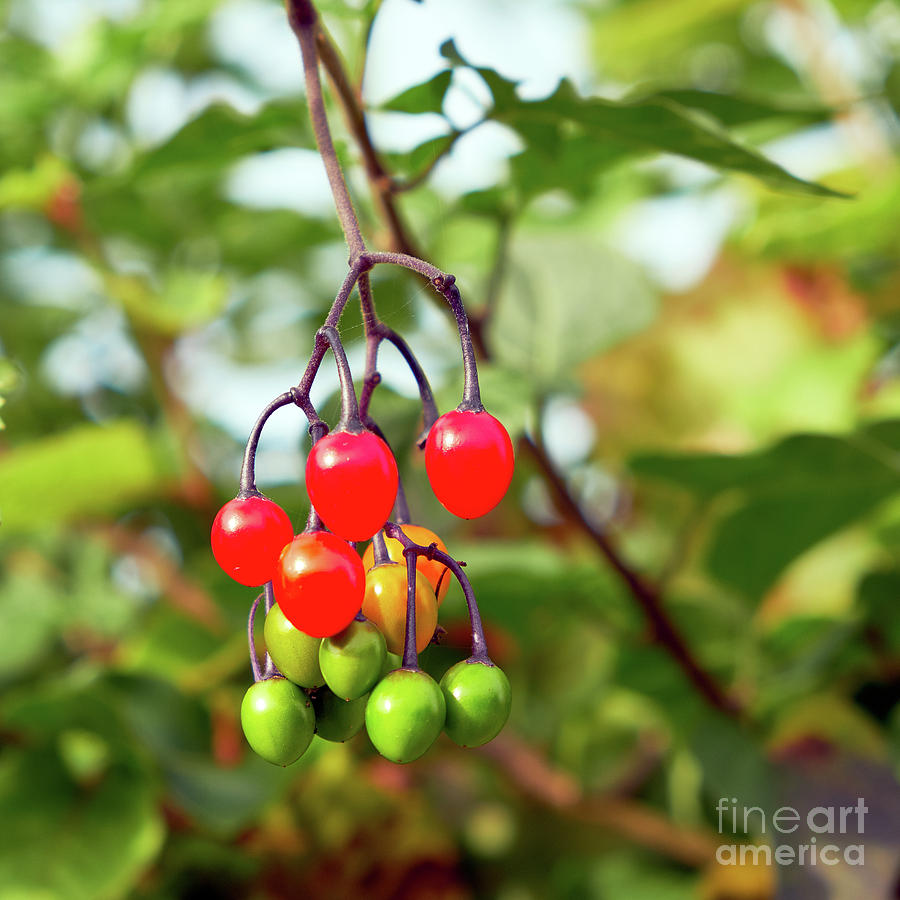This is a highly detailed, close-up photograph showcasing a cluster of berries hanging from a branch, likely from a tree or possibly a bush. The image captures these berries in various stages of ripeness, creating a vibrant spectrum of colors. At the top of the cluster, you see around four bright red, almost translucent berries with noticeable subsurface scattering of light. Just below, there are two to three berries transitioning through a light orange to yellow hue, exhibiting a high degree of reflectiveness but lacking translucency. At the base of the cluster, the berries shift to a deep green, reminiscent of green apples, with no translucency observed. The berries are individually connected by short dark brown stems that merge into a single main stem, from which the cluster hangs. The background is artistically blurred, featuring shades of green and hints of gold and orange, providing a beautiful, ethereal backdrop without revealing specific details of the setting. Notably, at the bottom right corner of the image, the logo 'Fine Art America' is displayed, marking the artwork's origin.